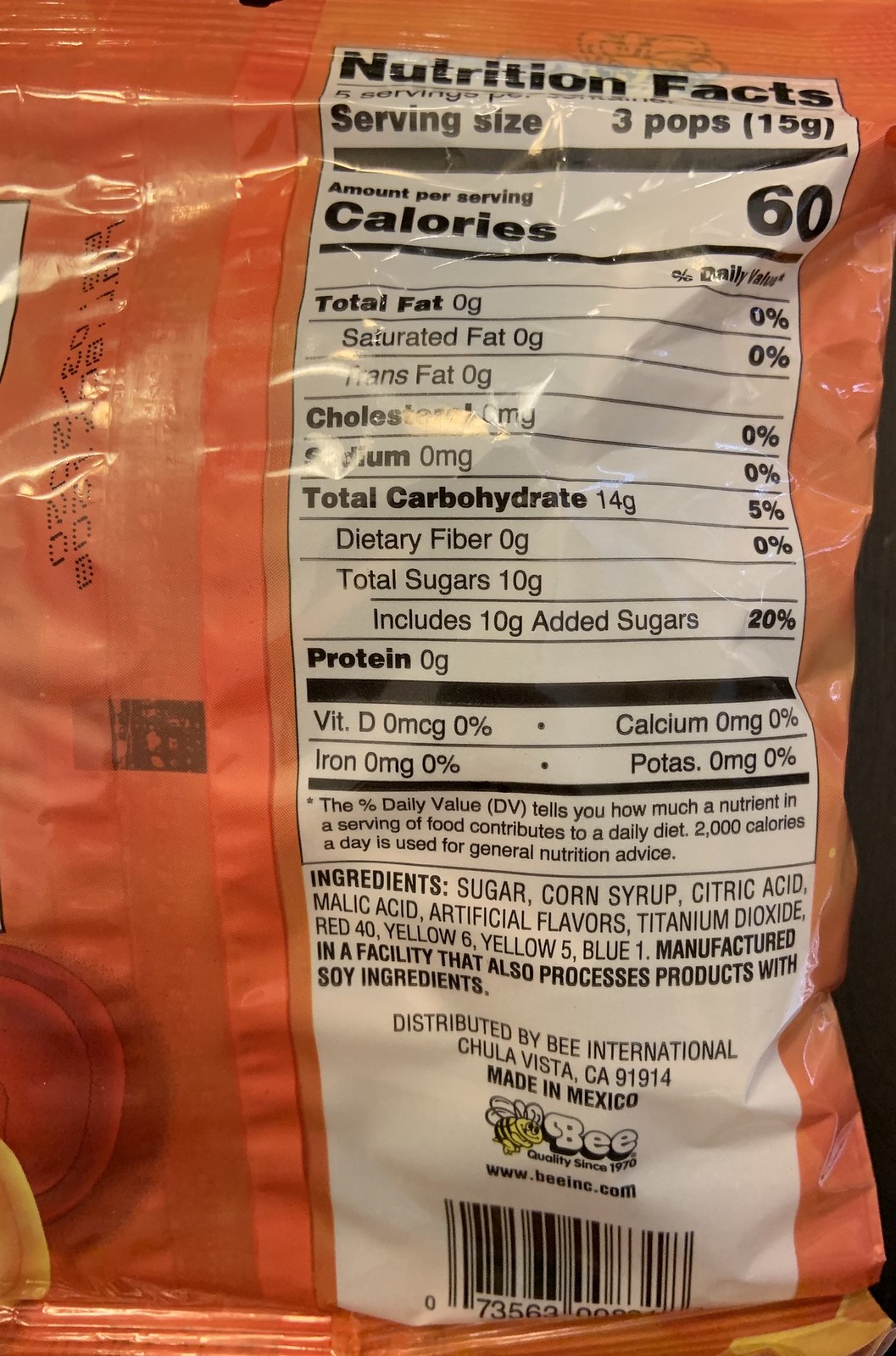This is an image displaying the nutrition facts label of an orange candy bag. The label specifies nutritional details for a serving size of three pops. Key nutritional values per serving include 60 calories, 0 grams of total fat, saturated fat, trans fat, cholesterol, and sodium. The total carbohydrate content is 14 grams, accounting for 5% of the daily value, with 0 grams of dietary fiber, 10 grams of total sugars, and 10 grams of added sugars, comprising 20% of the daily value. The candy contains no protein, vitamin D, iron, calcium, or potassium. 

The listed ingredients are sugar, cornstarch, citric acid, artificial flavoring, titanium dioxide, Red 40, Yellow 6, Yellow 5, and Blue 1. Additionally, the product is manufactured in a facility that processes soy ingredients. An expiration date is printed on the back of the bag, although it is not clearly legible in the image.